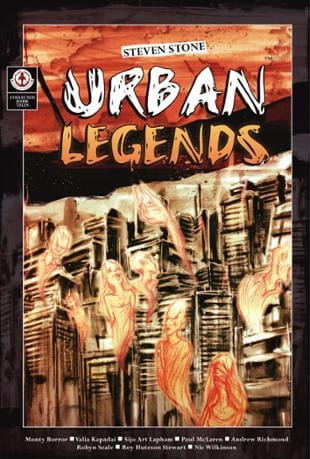The image appears to be a book cover, likely of a horror or urban fantasy genre titled "Urban Legends" by Stephen Stone. The cover is rectangular with a brown border and features Stephen Stone's name prominently at the top, slanted. The title "Urban Legends" is written in a graffiti-esque, rustic white and light orange font, both outlined in black. The top portion of the image depicts fiery red clouds against a dark strip, creating an eerie atmosphere. Below, an impressionistic cityscape of tall skyscrapers sketched in black and tan colors stretches upwards. Interspersed within the urban environment are ghoulish, ghost-like figures, some with orangey-red tints, adding to the haunting scenery. One prominent feature is an eerie hand emerging from the middle of the scene. Additional text is present at the bottom, but it is too blurry to discern clearly. Overall, the cover evokes a sense of supernatural urban mystery, possibly appealing to younger readers or fans of spooky tales.